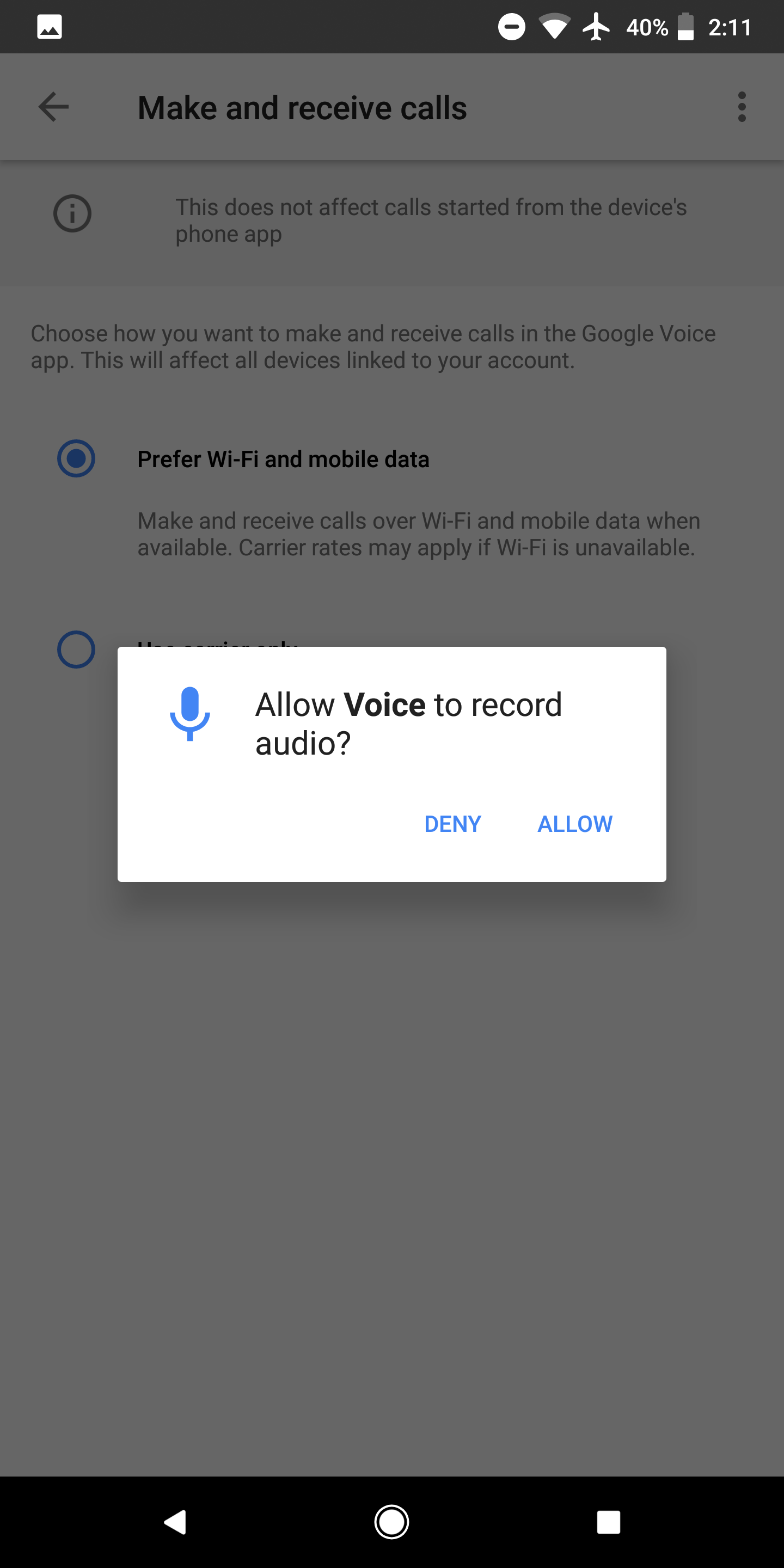In the image, a black telephone icon is positioned at the top left. Adjacent to it is a small white square containing two black dots. Below this is a white circle bisected by a black line, followed by a white arrow pointing downwards. An airplane icon is also visible, with "40%" displayed next to it, and the number "211" just below.

The background is gray and blurry, but underneath the aforementioned icons and text, there is a small circle with an eye symbol next to a message stating: "This does not affect calls started from the device's phone app. Choose how you want to make and receive calls on the Google Voice app. This will affect all devices linked to your account."

Further down, there is a small blue circle with an icon inside, labeled "Prefer Wi-Fi and mobile data." The accompanying text reads: "Make and receive calls over Wi-Fi and mobile data when available. Carrier rates may apply if Wi-Fi is unreliable."

Additionally, a white box contains a blue microphone icon, with black text asking, "Allow Voice to record audio?" Below this text, there are two blue options: "Deny" and "Allow."

At the bottom of the image, a black strip features a white arrow, a white round button, and a small white square.